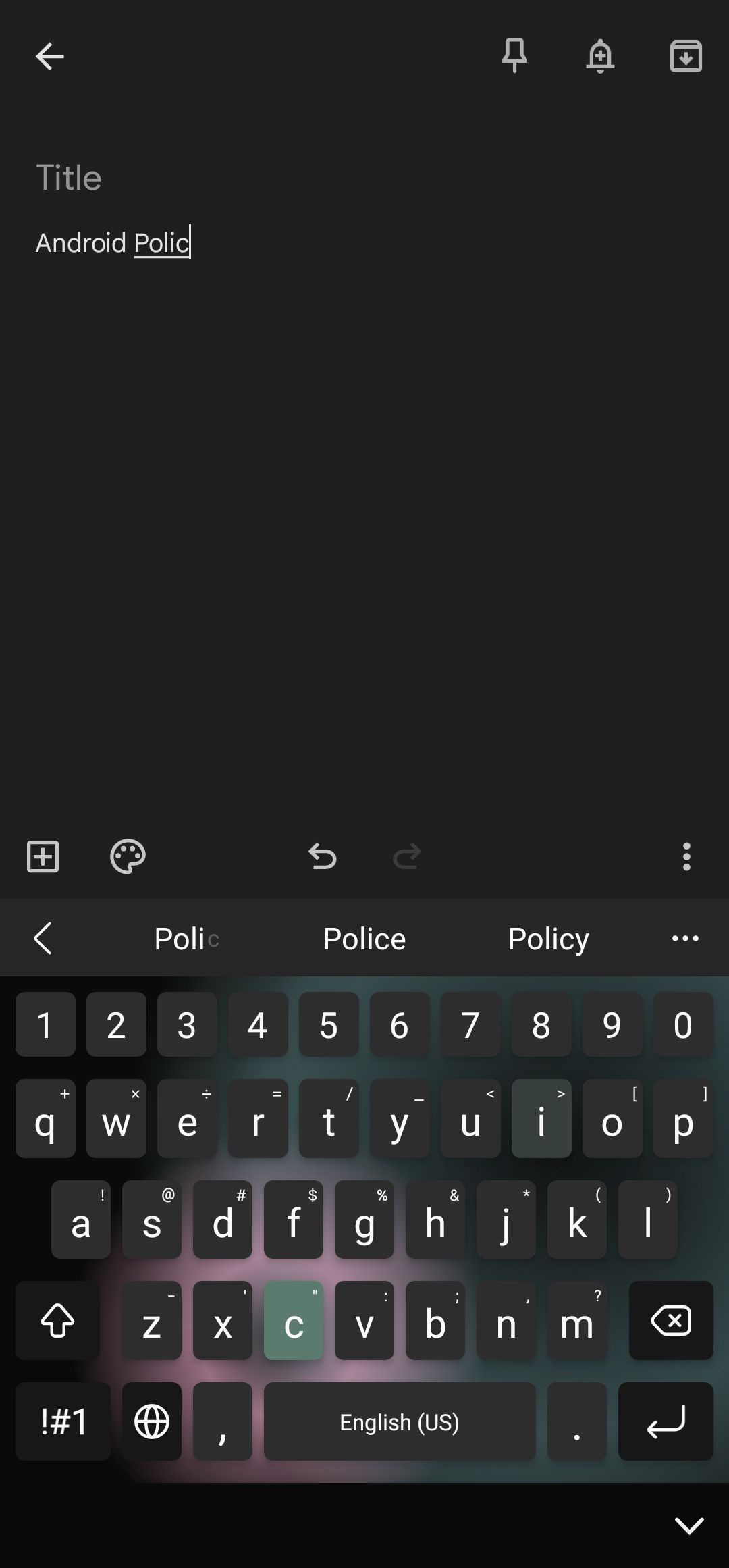This image is a screenshot from a mobile device interface. In the upper part of the screen, there is a left-facing arrow in the top-left corner and three icons in the top-right corner. Below this, the word "title" is displayed in gray, followed by the text "Android Pollock" (mistakenly typed as "P-O-L-L-I-C") separated by a vertical bar. The main section of the image is mostly black, occupying the top half of the screen. Below this area are several icons: a plus sign, an art palette representing color choices, a return icon, a grayed-out forward icon, and a three-dot menu indicator. 

Further down, we see suggestions related to the word fragment "P-O-L-I", with different options to complete the word. The fragment is displayed in bright highlight with "C" dimmed, followed by the options "police" and "policy". 

At the very bottom of the screen is a virtual keyboard. The top row shows numbers 1 through 9 and 0. The QWERTY letter arrangement follows, with the "I" key in a lighter shade of gray. The row below contains "A-S-D-F-G-H-J-K-L". The row under that includes "Z-X-C" with the "C" highlighted in green, followed by "V-B-N-M". Additional keyboard functions include a shift key, a backspace arrow, a button for special characters and numbers, a globe icon for language selection, a comma, the text "English (US)", a period, and a return/enter key.